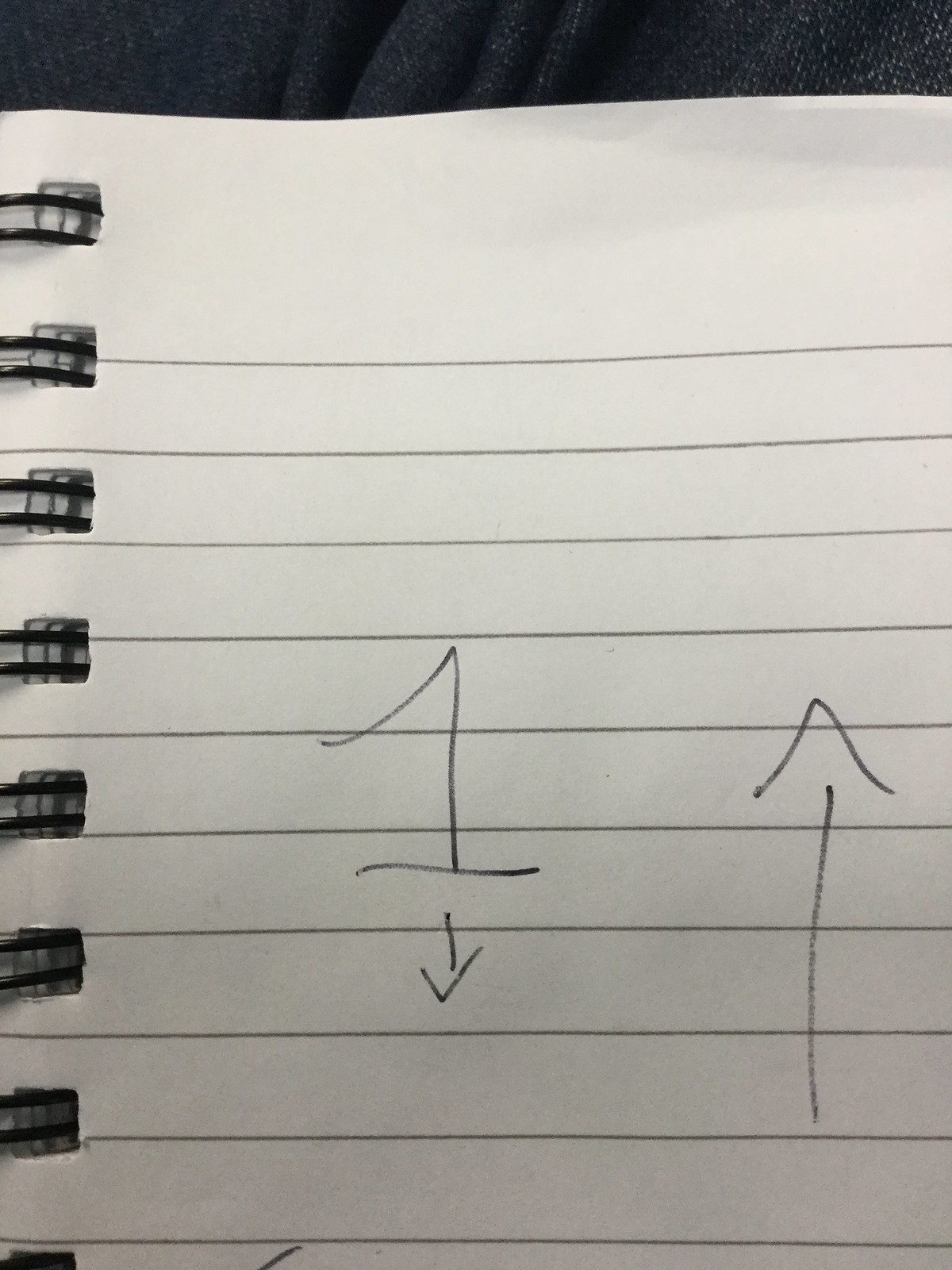The close-up portrait-oriented photograph showcases a spiral-bound notebook placed on a surface that resembles blue denim fabric. The notebook features white, lined paper with black spiral binding. Central to the image is a handwritten number "1" in black pen, accompanied by an arrow pointing downwards. On the right side of the page, there's another arrow, this one pointing upwards. The intricate details of the notebook and the texture of the blue fabric provide a tactile quality to the composition, capturing just a small portion of the notebook in this detailed close-up.